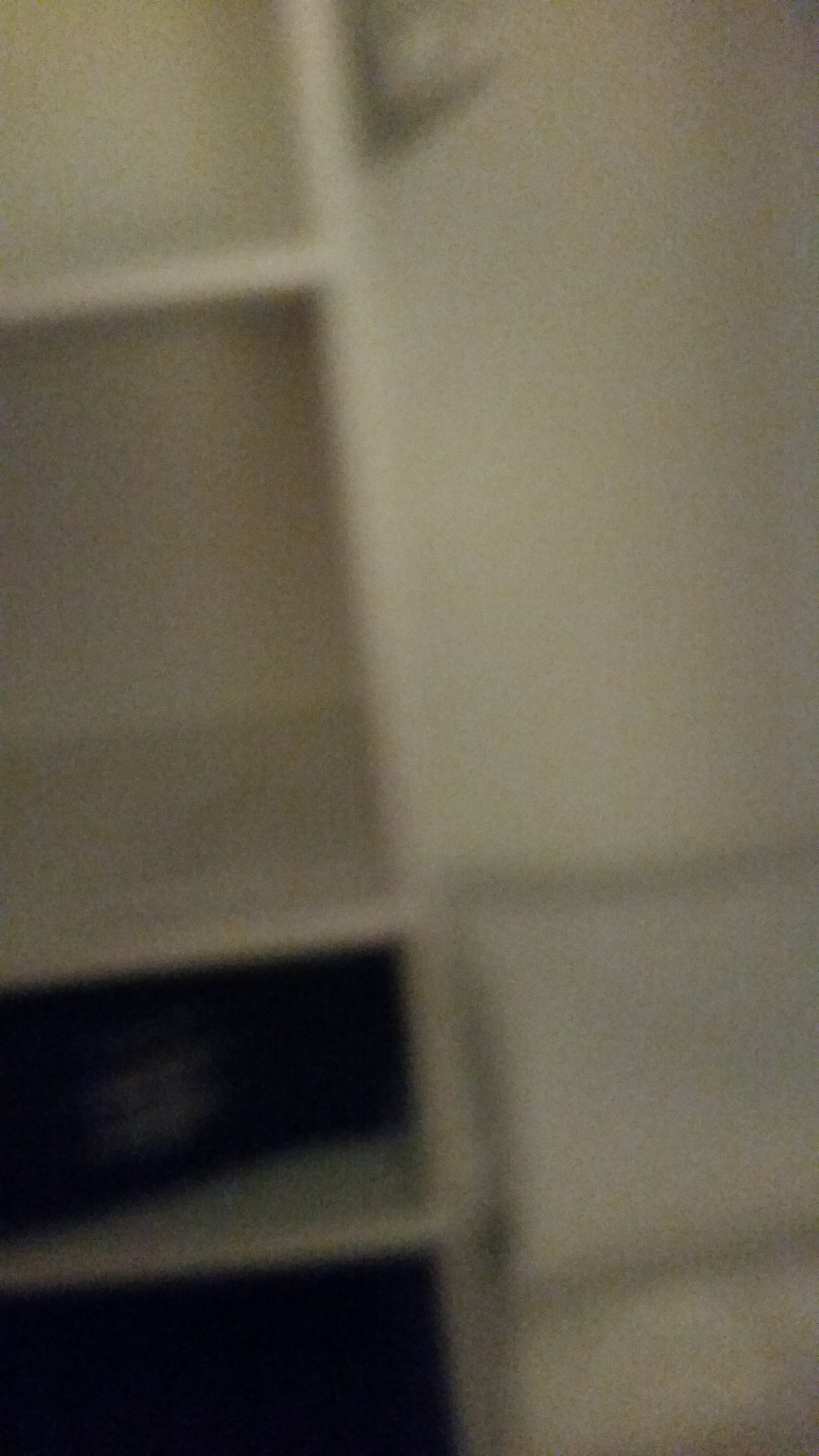The image is a somewhat blurry digital photo taken indoors, showing a white cubby-like shelving unit on the left side and a white wall with a square pillow on the right. The shelving unit has four open sections, with the top two being larger than the bottom two. The middle section appears to be the biggest. The interior of the lower shelves look darker, possibly due to shadows or the presence of black objects. On the bottom right, a bed with a white bedspread is partially visible. To the right, about three-quarters down, a white square pillow is propped against the white wall. The bottom right side of the image features a white curtain with visible seams forming three sections.